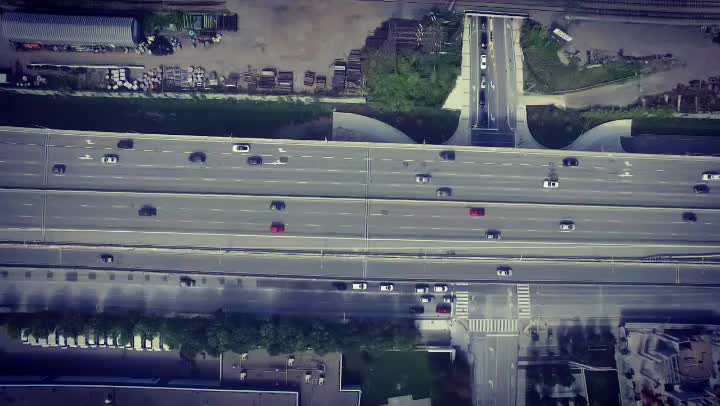This aerial image captures a bustling urban freeway from a top-down perspective. The freeway features four lanes in each direction, running east and west, filled with cars of various colors, including red, white, dark gray, and black. The scene also includes an overhead bridge crossing the freeway, beneath which is a secondary road running vertically, also populated with vehicles. Surrounding the freeway and the secondary road are lush green trees and bushes, adding a touch of nature to the urban landscape. The freeway itself is intersected by a road below, complete with crosswalks marked by white lines, where cars are waiting at the intersection. Additionally, parked cars are visible near the roadways, along with various buildings and a notable concrete area at the top of the photo, seemingly a construction site with stacks of pallets and an adjacent large, empty lot.